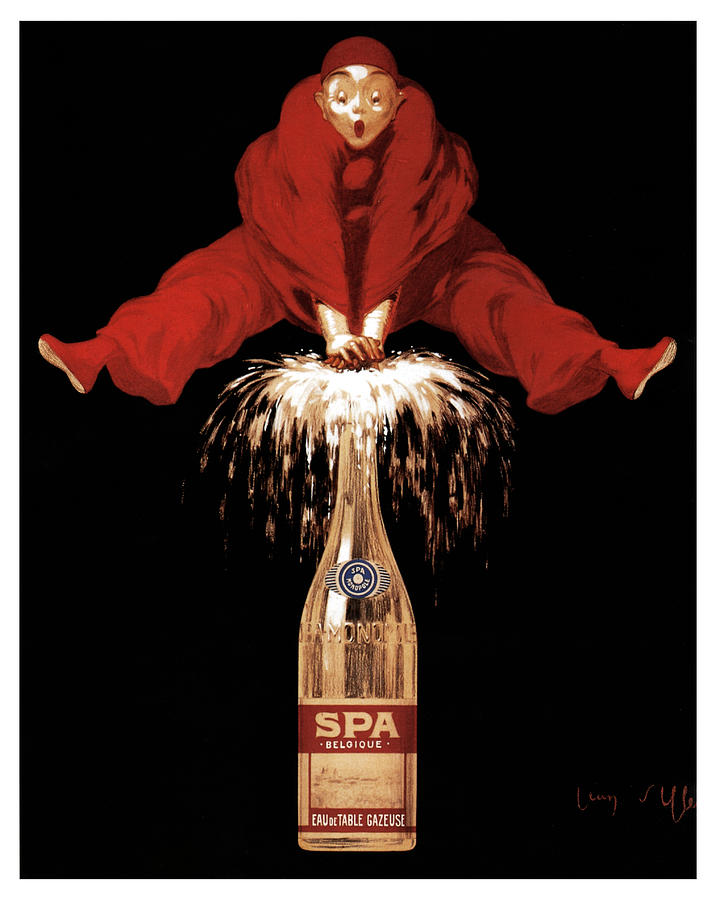In this vibrant, painted illustration, we see a striking scene set against a solid black backdrop. Dominating the image is a large, bright gold champagne bottle labeled "Spa Belgique" with additional indecipherable text in smaller fonts below. Emanating from the bottle's top are explosive, firework-like streams of champagne. Perched atop this effervescent display is a figure dressed entirely in red, including a red skull cap and shoes, with a look of astonishment on his face. He appears to be a French clown or Pierrot executing a handstand on the champagne burst. The detailed, square-shaped painting also features a small, light orange, cursive artist's signature in the bottom right corner, adding a final touch to this whimsical and dynamic composition.